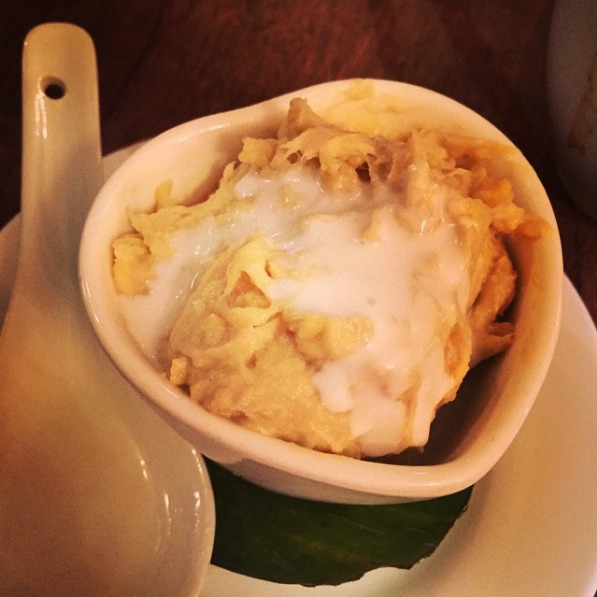A yellow, possibly starchy food resembling mashed potatoes or pasta with a white sauce is elegantly served in a heart-shaped ceramic bowl. This bowl, which appears to be orange-colored or ivory based on differing descriptions, rests on a green leaf, all of which is presented on a round white ceramic plate. To the left of the bowl, there is a white porcelain soup spoon with a circular hole at the top. The entire arrangement sits on a brown table that is visible near the top of the image. The white sauce contrasts distinctly with the yellow coloration of the dish, creating a visually appealing presentation.